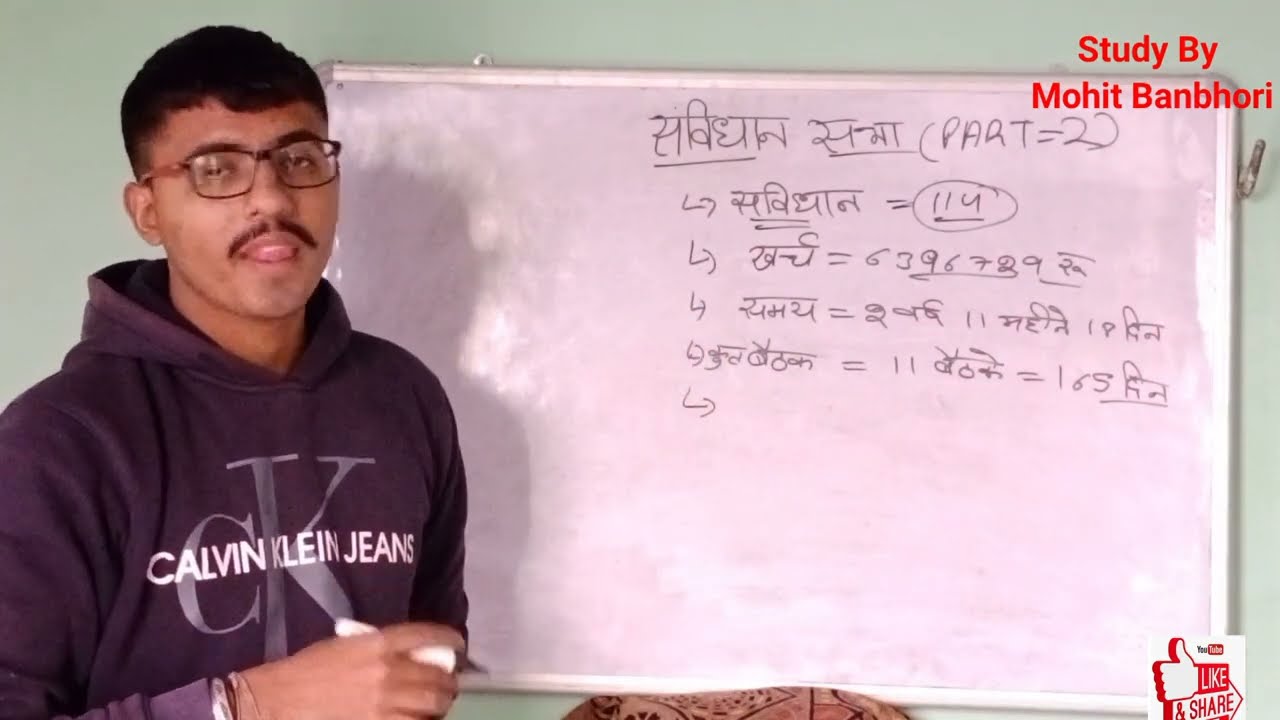In the image, a young Indian man stands in front of a small, well-used whiteboard mounted on a very pale green wall, almost off-white. The man has light brown skin, dark brown hair, a mustache, and wears glasses. He is caught mid-lecture, half-blinking as he appears to be speaking, holding a dry erase marker in his right hand. The man is dressed in a distinctive purple Calvin Klein jeans hoodie, which has the brand's name and 'CK' logo on it. The whiteboard behind him features a mix of unreadable characters, possibly Sanskrit, along with some numbers and the phrase "part two." The image looks like a screenshot from a YouTube video, emphasized by red text in the upper right corner stating "study by Mohit Banburi," and a prompt in the lower right corner saying "like and share."